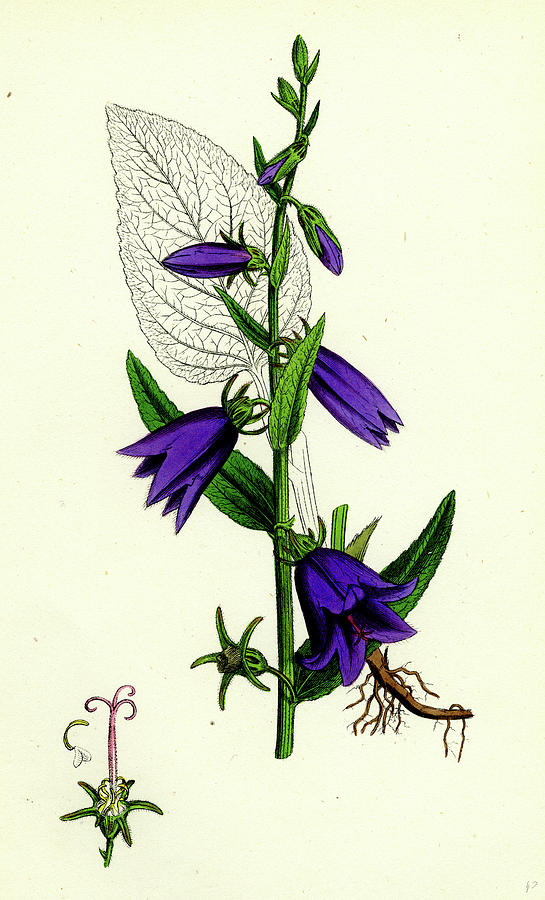The image is a highly detailed, color hand-drawing of a botanical specimen on light beige paper. The focal point of the artwork is a tall, thick green stalk adorned with big, pointy leaves. Distinctively, some of these leaves appear lace-like, showcasing intricate vein structures without any green tissue. The plant features several bell-shaped flowers that transition from small, closed buds at the top to fully opened large blooms at the bottom. These flowers, dark purple in hue, bear a resemblance to tulips but with a form more akin to daffodils, and they include a red stamen at their centers. Complementing the main illustration are additional elements: a detailed stencil sketch of a leaf's veins in the background, a pink protrusion encircled by leaves in the lower left corner, and a section of brown plant root in the lower right, completing the botanical depiction.